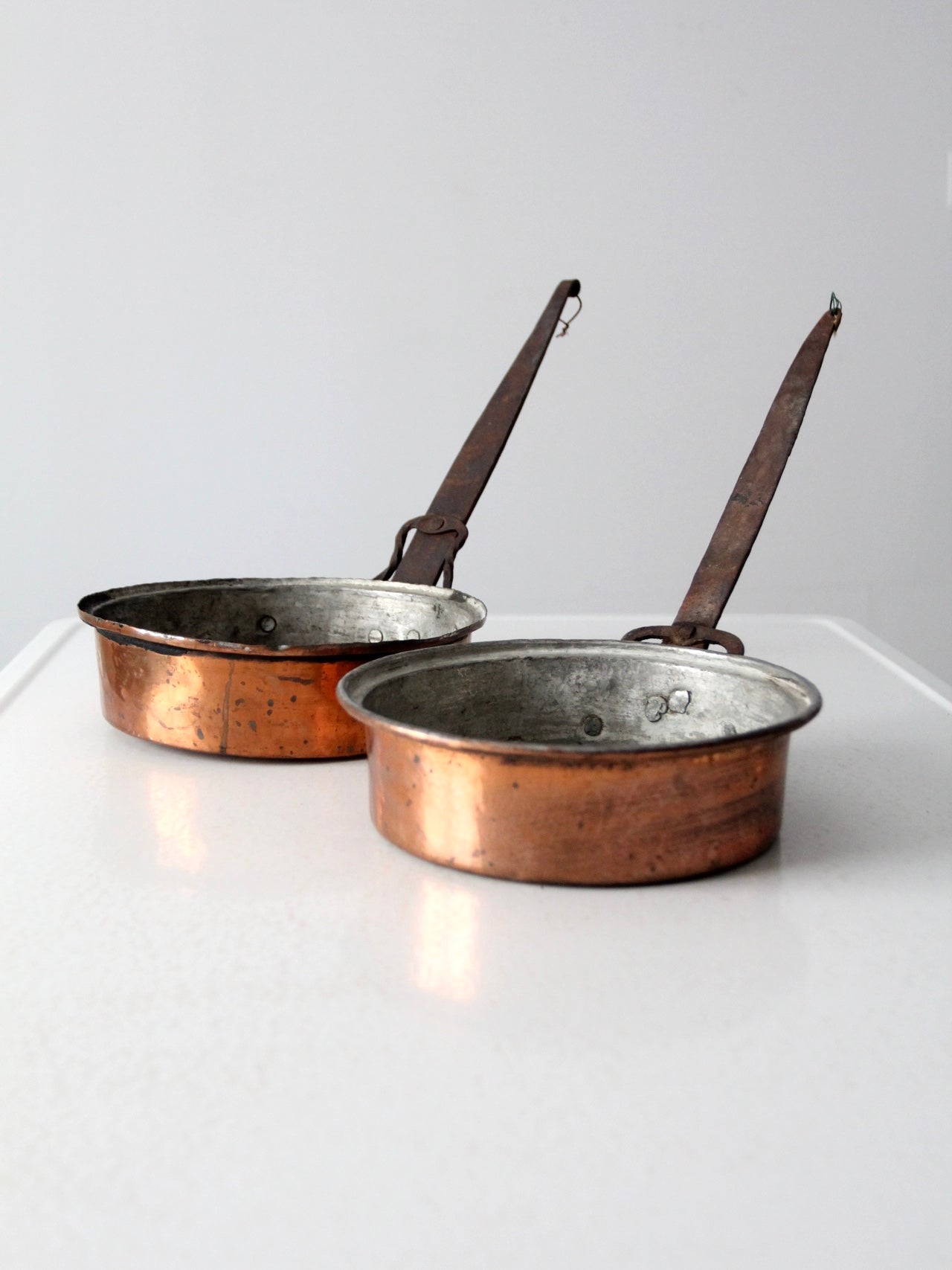The image depicts a vertically aligned rectangular photograph of two old, weathered copper pots placed on a white countertop with slight raised edges on the sides. The background is a light gray wall, providing a simple, unobtrusive backdrop that emphasizes the aged cookware. The copper pots themselves are heavily worn, with numerous dark gray markings on their silver-colored interiors and speckled white and black dots and streaks on their copper exteriors. Each pot has a handle that extends outward at an approximate 45-degree angle, with the handles showing significant rust and little strings hanging from their tips. The handles, likely made of iron, are attached to the pots by screws and feature welded dots visible on the inside metallic surface. These handles taper to a point and curve slightly downward at the end. The overall scene captures the rustic charm and longevity of these vintage cooking essentials.